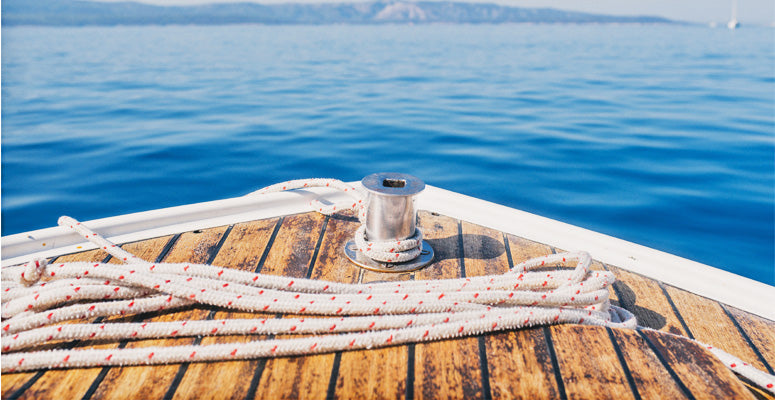This is a detailed up-close photograph of a lake, with the opposite shore forming a thin strip of land at the very top of the image. The water is a gradient of blue, with a rich, royal blue at the center gradually lightening towards the horizon. In the foreground, we see the front of a boat shaped like an upside-down ‘V’. The boat has a white border and rustic brown wooden flooring. Lying horizontally across the deck is a white rope adorned with reddish-orange dashes. Near the point of the boat, in the center of the image, is a silver or chrome cleat where the rope should be wrapped around, although most of it remains loose on the deck. The water is strikingly blue, and there are hints of other boats or objects in the blurred, distant background. This picturesque scene showcases the tranquility of the lake juxtaposed with the functional details of the boat’s deck.